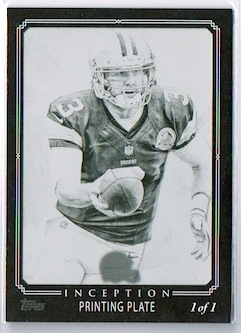The image depicts a trading card encased in a clear acrylic protective case, visible along the card's borders. The card features a black border with a white inner border, framing a black and white photograph of a male football player. The player is wearing a black or gray jersey with the number three near his shoulder pads, white pants, and white gloves. He sports a white helmet with two white stripes running down the center. The player is mid-catch, holding a football in his right hand while his other hand is outstretched. The card has multiple lines of white text; "T O P P S" appears in the bottom left corner, "Inception" is centrally placed, and "Printing Plate" is towards the bottom right corner, accompanied by the text "One of One." The entire card is set within a black background, and the acrylic case provides an additional layer of protection that is noticeable around the card’s edges.